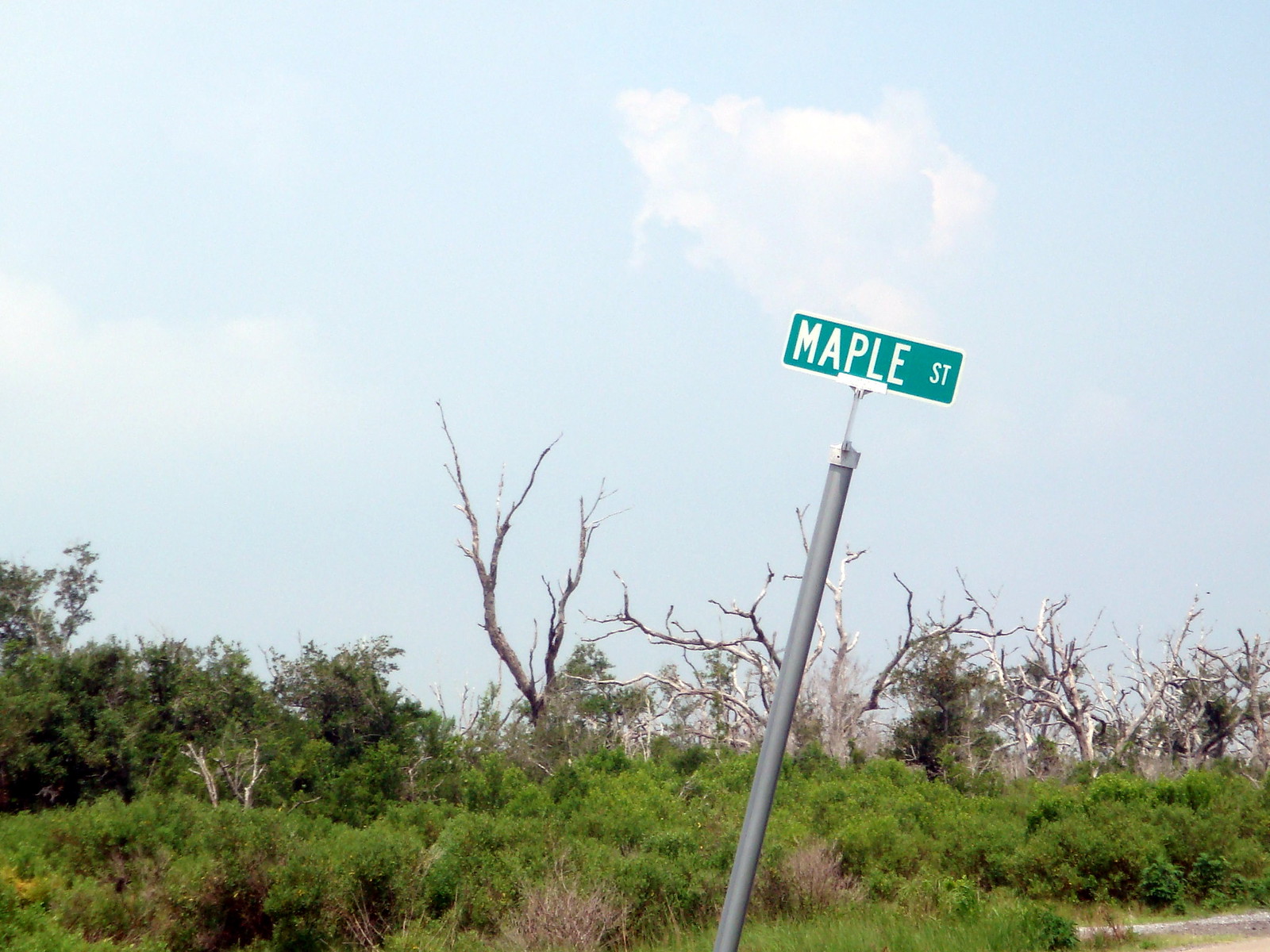This photograph captures a bright, sunny afternoon with a clear, light blue sky dotted by scattered puffy clouds. The background reveals a dense mix of trees and bushes, including several dried-out, leafless, and broken trees indicating a lack of recent maintenance. In contrast, the foreground is filled with untamed foliage and high bushes, further emphasizing the natural, unkept environment. Positioned towards the middle-right of the image, a metal gray street post stands out, tilted slightly to the right at its top. At the summit of the post is a green sign adorned with white letters, clearly displaying "Maple Street."